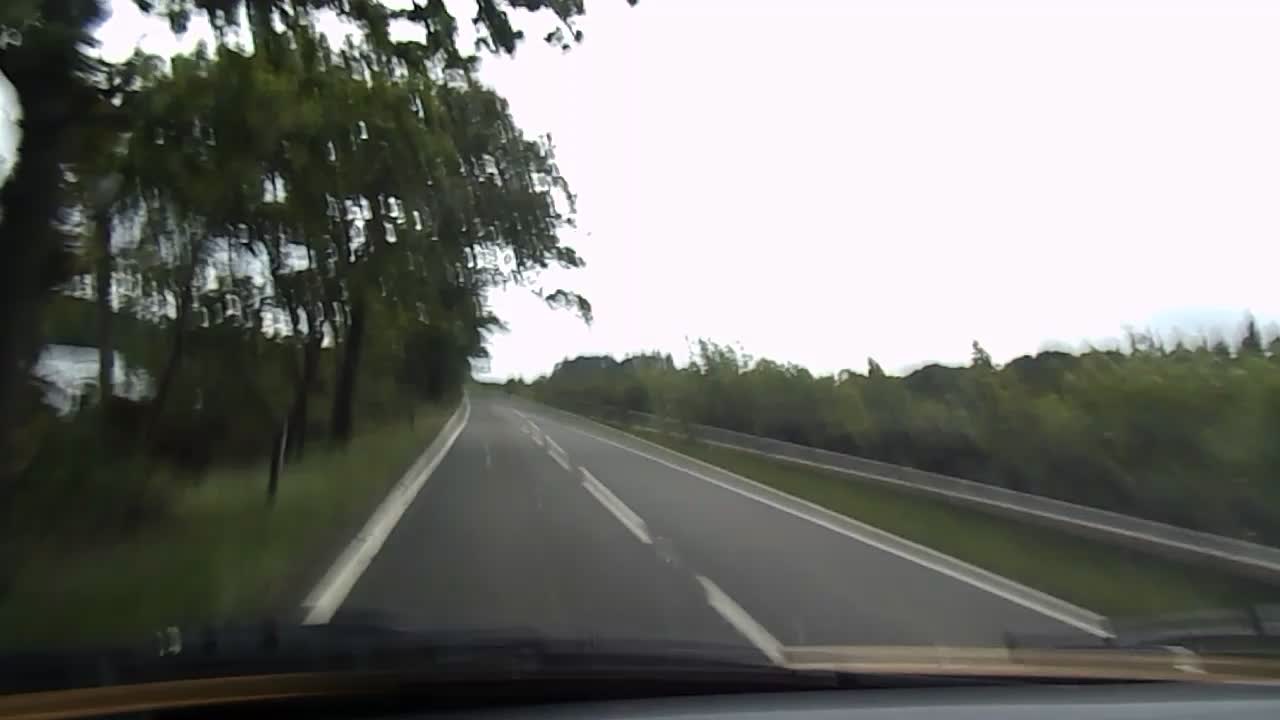A serene photograph captures the experience of driving on an empty highway from the front seat of a car. Windshield wipers are faintly visible, hinting at a recent rainfall. The vehicle is traveling on the left side of the road, indicating that this scene likely takes place in a country where left-hand traffic is the norm. The road is lined with dashed center lines and solid edge lines. To the right, a sturdy guardrail separates the highway from a dense expanse of trees, while a similar tree line flanks the road to the left. The road ahead is noticeably devoid of other vehicles, creating a sense of solitude and open space. The photograph is bathed in light, rendering the sky an almost white hue, which adds to the overall calm and airy atmosphere of the scene.